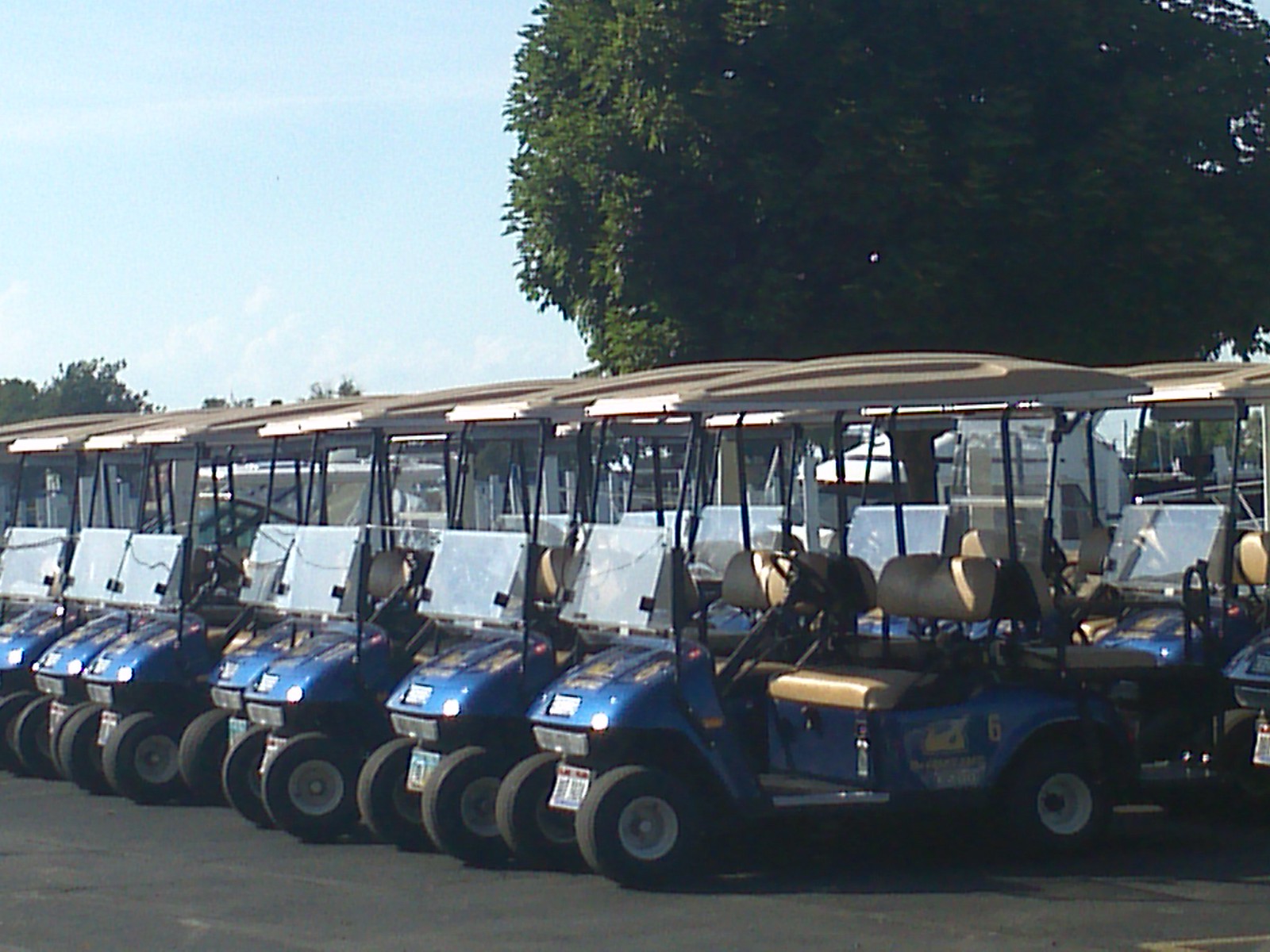The image captures two visible rows of nearly identical golf carts neatly lined up on black asphalt. Each golf cart features a deep blue frame, a tan hard plastic canopy, and tan bench seats with the rear seat facing backward. The carts are equipped with black rubber tires with white rims, and a fold-down windscreen currently positioned downwards. License plates are affixed to the front of each cart. The background reveals a single, large deciduous tree with a rounded, dense canopy of dark green leaves, and the pale green sky creates a slight haze with some visible glare, adding to the scene's natural lighting. Just above the canopies of the golf carts, the tops of additional trees can be seen. Although the first row contains six or seven golf carts, the number of rows and carts further back remains unclear.